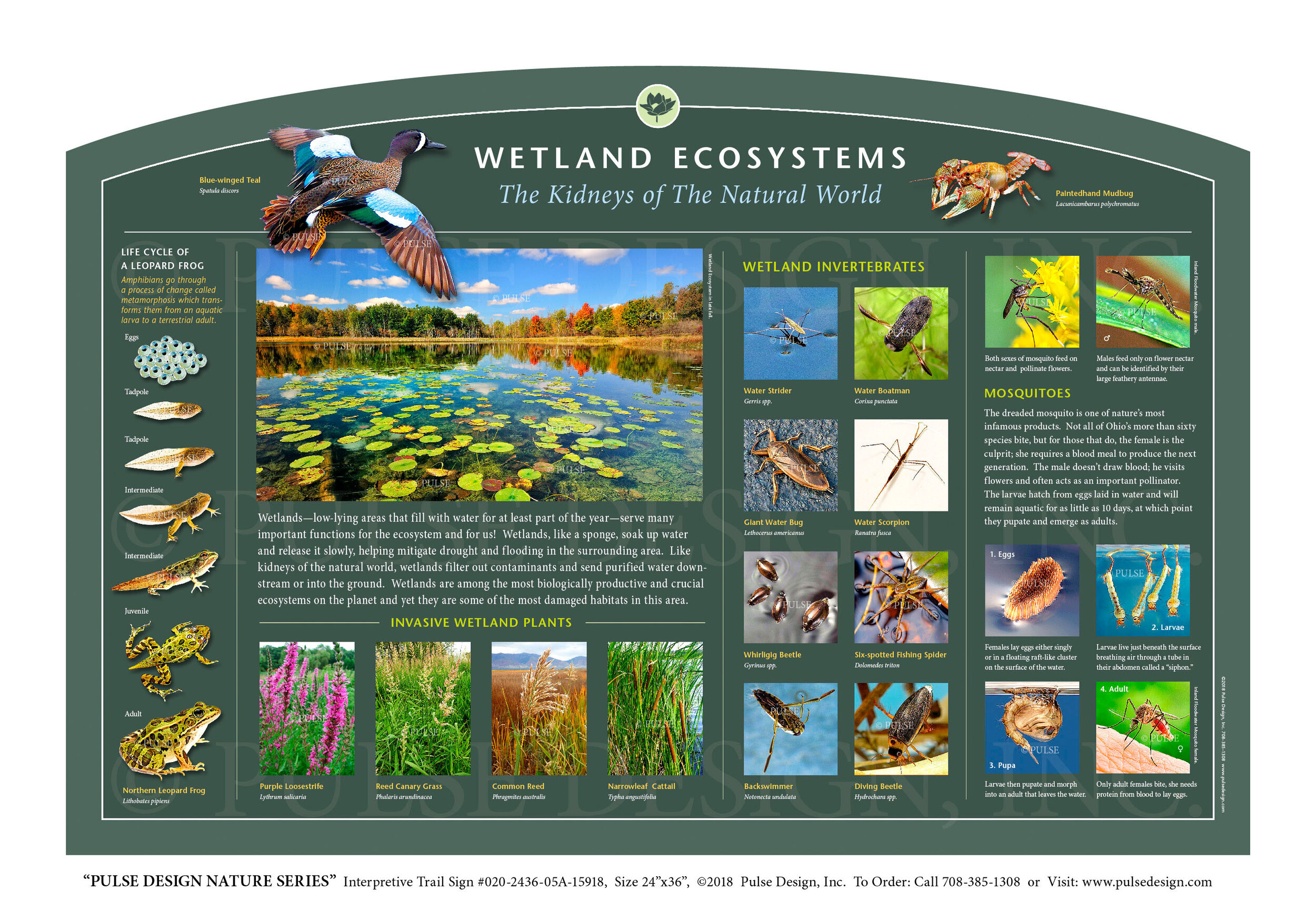This educational image, likely a billboard from a natural park, is titled "Wetland Ecosystems: The Kidneys of the Natural World." It features a rich array of detailed information and images about various wetland inhabitants and their life cycles. Dominating the top section are photographs of diverse wetland creatures, including a mallard duck on the left and what appears to be a lobster on the right. The most prominent image shows a picturesque marshland with a lotus flower in the foreground and a forest in the background.

To the left, a detailed series of images portrays the life cycle of a leopard frog, from eggs and tadpoles through to the intermediate stages and culminating in the juvenile and adult frog. Below, sections are dedicated to different categories, such as invasive wetland plants, depicted with four distinct images, and wetland invertebrates, with eight labeled pictures showcasing species like water striders, water boatmen, giant water bugs, and water scorpions. Additionally, there's information on mosquito life cycles, complete with images illustrating their stages from eggs to pupae.

The bottom of the sign reads "Pulse Design Nature Series Interpretive Trail Sign," providing information about the production and availability of the sign for educational purposes. This comprehensive and visually engaging presentation offers an in-depth look at the vital roles and various life forms within wetland ecosystems.